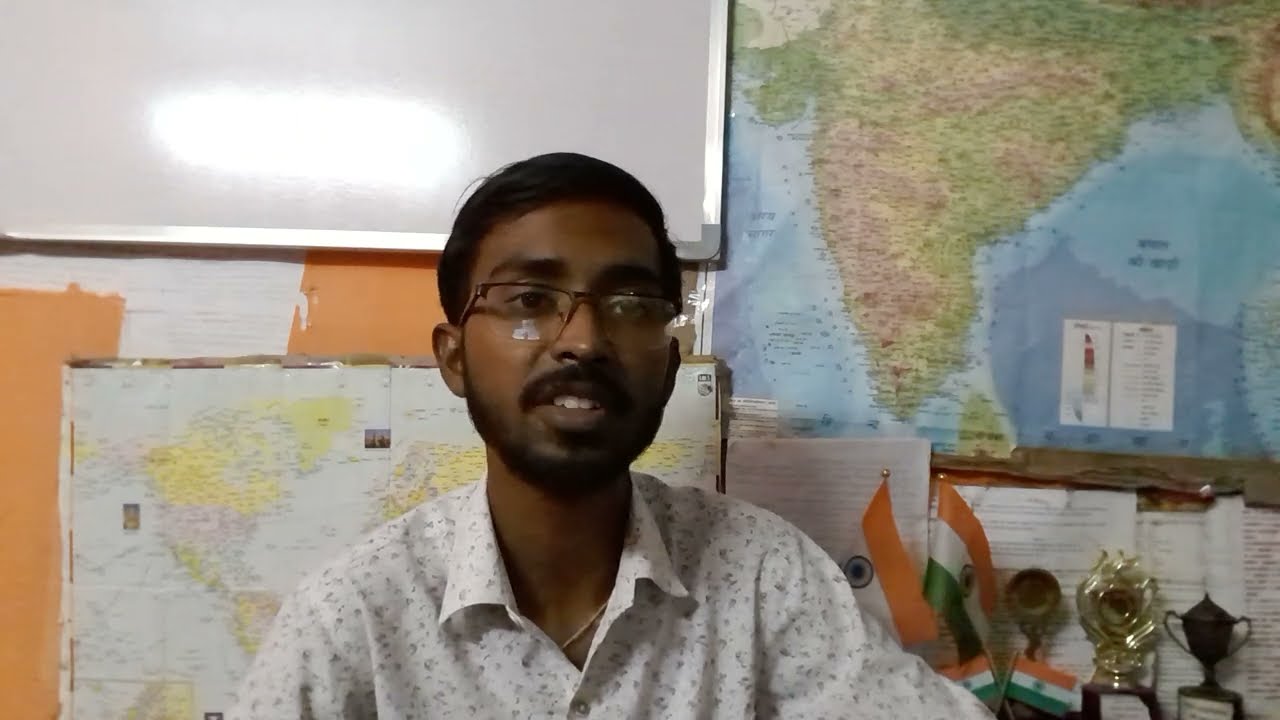This image features a dark-skinned man, possibly of Indian or Arabic descent, sitting in what appears to be a classroom or office environment. He has a thin build, round head, and dark brown-black hair parted at the temple and swept to the left. The man has thick black eyebrows, a mustache, and a beard extending underneath his chin. He is wearing glasses with wire rims on the top and an open bottom, and his mouth is open, revealing his upper teeth and full bottom lip. He is dressed in a long-sleeve, white button-up collared shirt adorned with gray patterns, possibly squiggly marks, triangles, or diamonds, and he accessorizes with a gold chain necklace.

The background includes a large map of Africa prominently displayed on the right-hand side of the image, with a whiteboard below it. Further to the left is a flat map of the United States. The wall beneath the whiteboard is orange. There are trophies and ribbons above the whiteboard, along with a few small flags featuring an orange, white, and green banner with a dark circle at the center of the white section. These details suggest this man might be in a professional or academic setting, possibly a professor. The image captures him talking to the camera, making it likely that this is a still from a video.